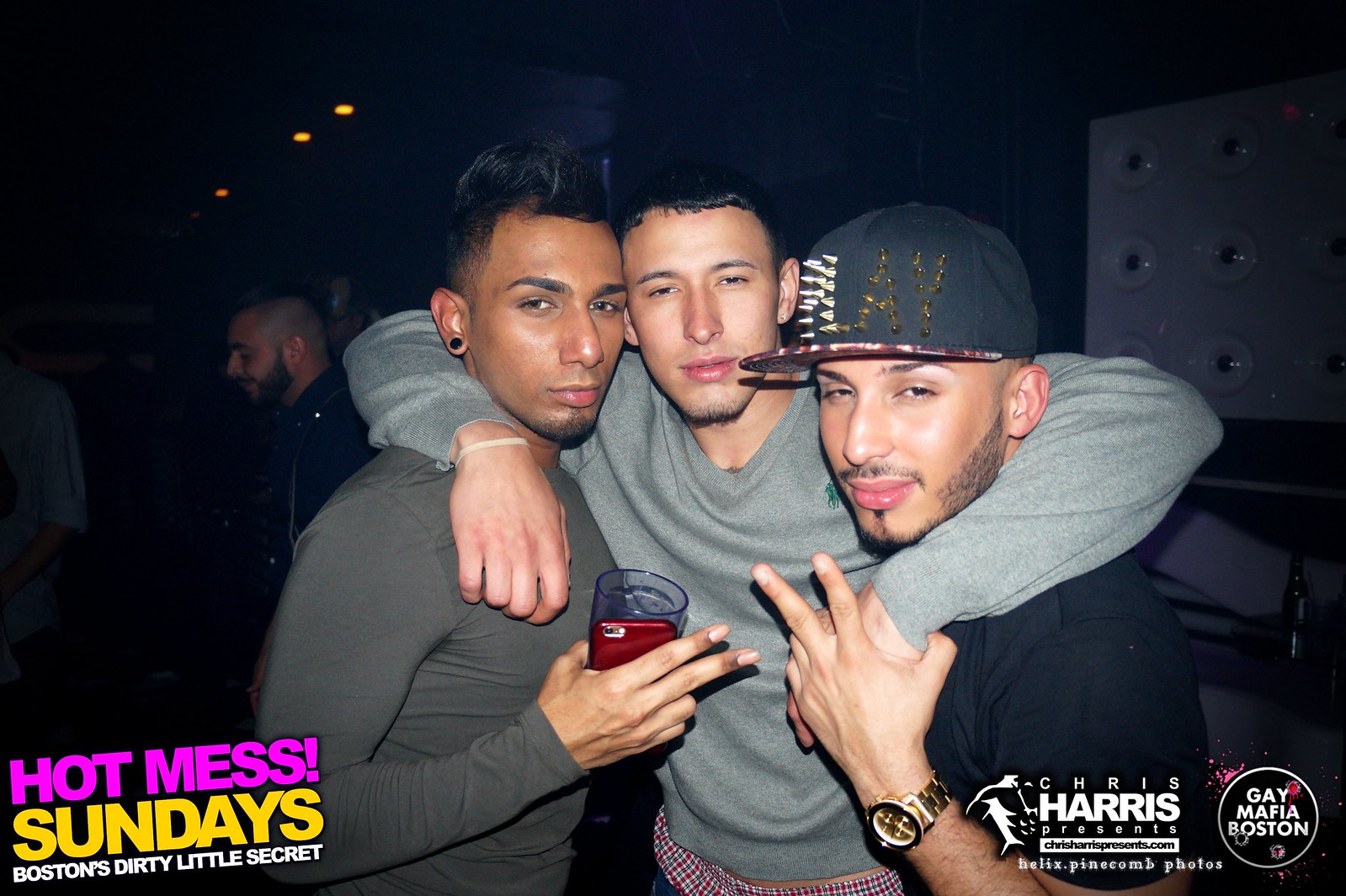In this rectangular photograph, three young men, likely in their early to mid-20s, pose closely together, with smiles on their faces, and the ambiance suggesting a nightclub setting. They're shown from the waist up. The man on the left sports a long-sleeved dark gray shirt and is holding a drink in one hand and a red telephone in the other. The man in the middle wears a light gray long-sleeved shirt, and the man on the right, who is in a black short-sleeved t-shirt, completes the group and is distinguished by a baseball cap and a gold watch.

The background is dimly lit, characteristic of a club, with bright overhead lights faintly visible, and a few other people can be seen mingling in the shadows. The setting is lively with an inviting hint of chaos.

Overlaying the bottom left corner of the photograph in bold hot pink text are the words "Hot Mess," followed by "Sundays" in yellow, and underneath that, "Boston's Dirty Little Secret" written in white. The bottom right-hand corner displays two logos. The first, a small graphic resembling a shark or fish, reads "Chris Harris Presents," and below it is an obscured website, likely "christharrispresents.com." Beneath this, the text "Helix Pinecone Photos" is evident. Adjacent to this is a circular logo with the text "Gay Mafia Boston" inscribed in white, marking the image as a promotional material, most probably for a gay nightclub event.